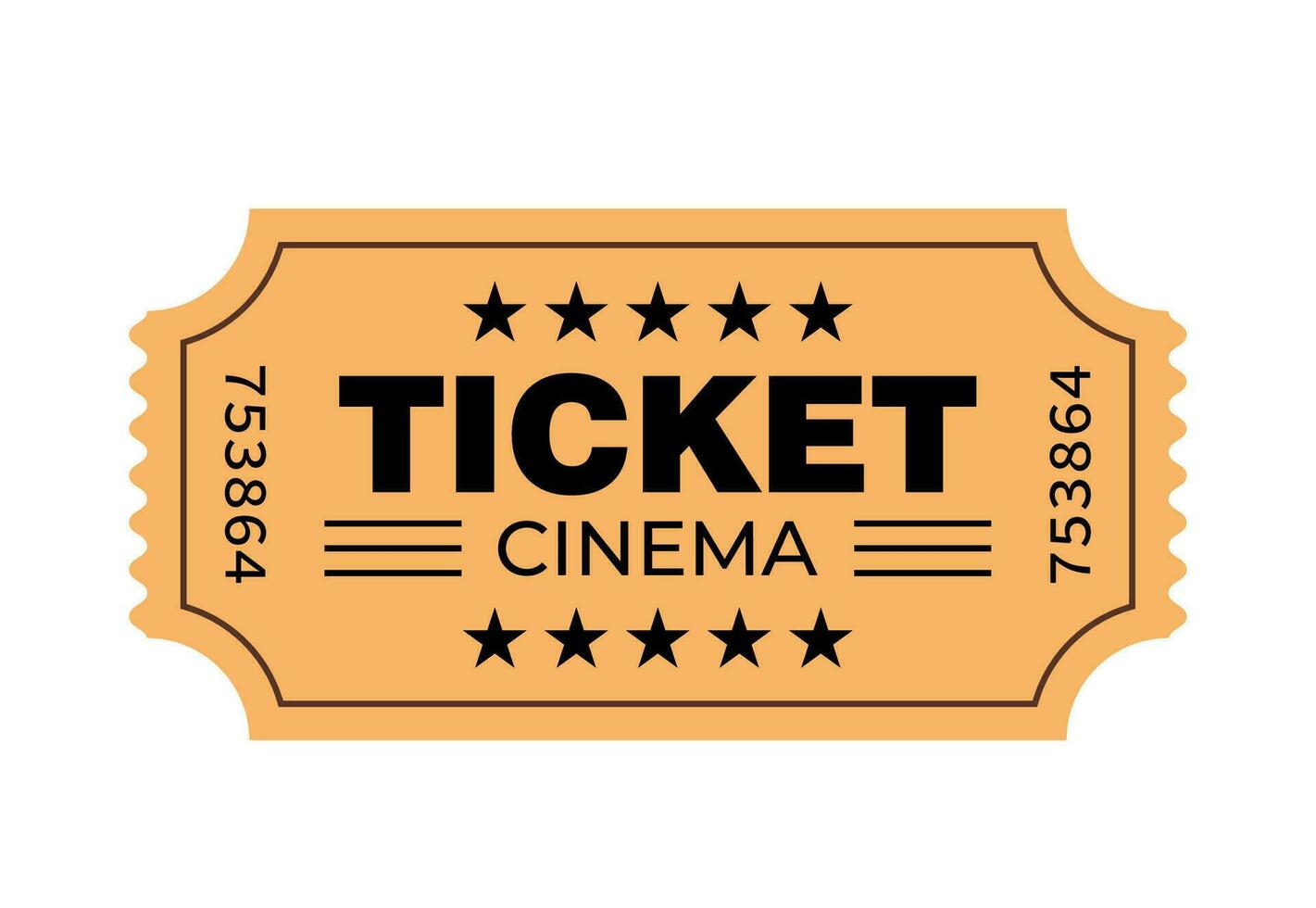This detailed description synthesizes elements from all three captions, providing a vivid and comprehensive depiction of the carnival ticket:

The image depicts a computer-generated carnival ticket with a distinctly vintage aesthetic, reminiscent of those from past movie theaters. The ticket has a yellow-orange, sherbet-like background, edged with a thin black border. The design features concaved corners, giving it an inset, arch-like appearance. The left and right sides of the ticket have perforated edges, suggesting it was torn from a roll of tickets.

On the top and bottom of the ticket, five black stars are evenly spaced, adding to its classic appeal. In the center of the ticket, large black text reads "TICKET," with "CINEMA" in smaller, thin black text directly below it. Flanking this central text are three horizontal lines on each side.

Oriented vertically along both the left and right edges, the number 753864 is printed in black, reinforcing the ticket's authenticity. The overall appearance of the ticket is more illustrative than photographic, suggesting it is a digital rendition intended for display on a sales website or similar platform.